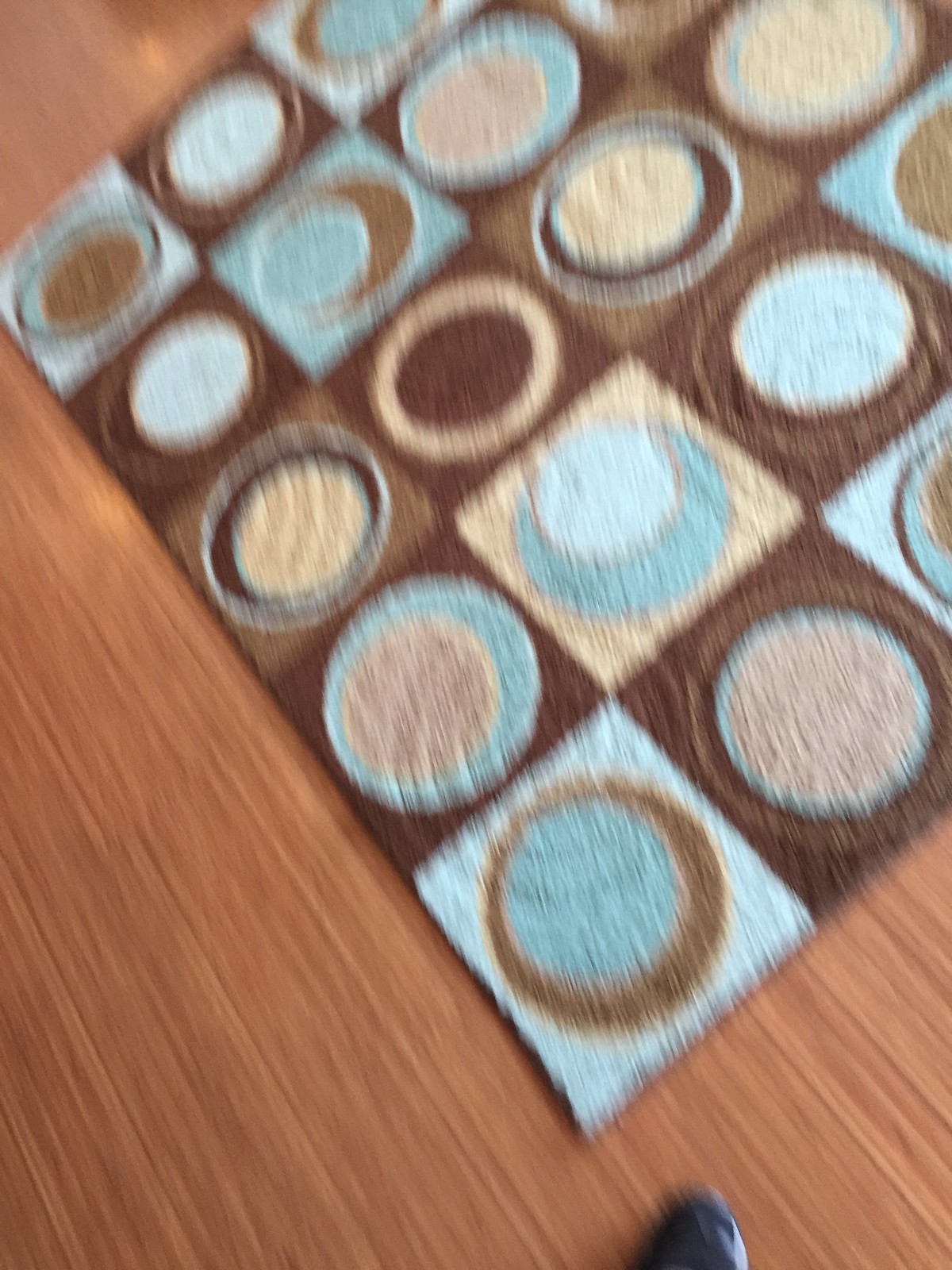A motion-blurred image features a vibrant rug styled from the 60s or 70s era. The rug showcases a grid pattern composed of various colors, with each square containing concentric circles in a palette of yellows, oranges, browns, and tans. The dynamic design rests on a medium to light-colored hardwood floor, or flooring that mimics this appearance. The lower portion of the image captures the cut-off view of the tail end of someone's shoe, adding a human element to the scene.